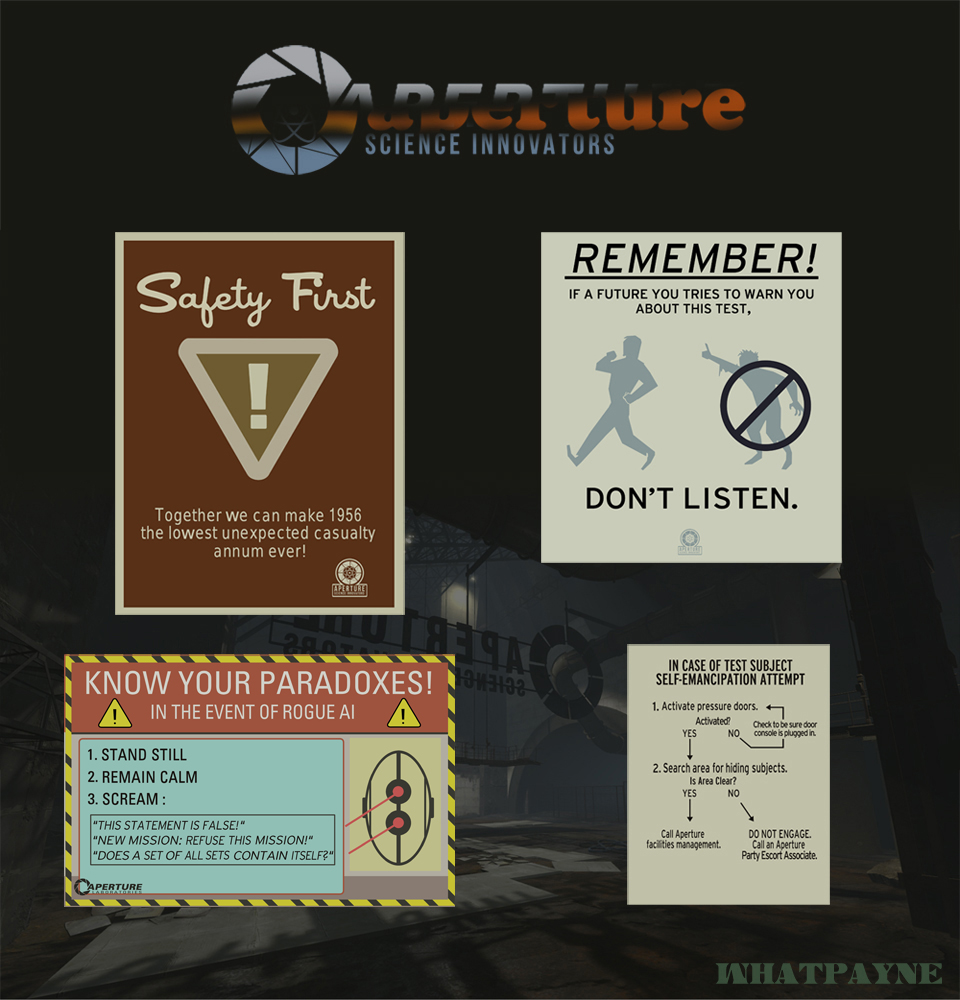The poster is a blackboard titled "Science Innovators" at the top in white, with a distinctive "O" encircled by lines and a red streak running from left to right. The board features four distinct safety-themed sections, each in a different color scheme:

1. **Safety First** (burnt brown with taupe lettering): This section features a yield sign with an exclamation mark and reads, "Together, we can make 1956 the lowest unexpected casualty annum ever."
   
2. **Future Warning** (taupe with black lettering): Depicts a man walking and another version of himself giving a warning, crossed out with a do-not-enter symbol. The text advises, "Remember, if a future you tries to warn you about this test, don't listen."

3. **Know Your Paradoxes in the Event of a Rogue AI** (multi-colored with yellow and black stripes): This section lists paradoxical instructions:
   - "1. Stand still."
   - "2. Remain calm."
   - "3. Scream."
   It also includes confusing statements such as "This statement is false" and "Does a set of all sets contain itself?"

4. **In Case of Test Subject Self-Emancipation Attempt** (grayish white): Details steps for containment involving activating pressure doors and searching the area for hiding subjects, with specific instructions on calling the appropriate facilities or party escort associates.

The board uses a mix of colors and visual elements like yield signs, exclamation marks, and crossed-out figures to deliver its safety messages in a creatively engaging format.